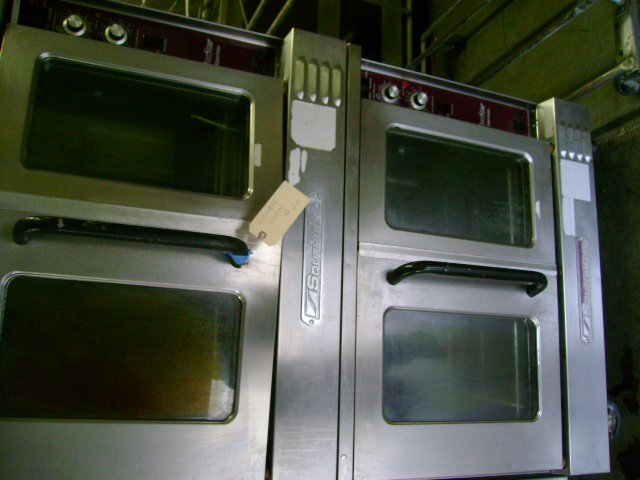This color photograph depicts an industrial kitchen setting featuring two large, stainless steel convection ovens made by South Bend. Each oven sports a long, black metal handle positioned in the middle of its double glass-paned doors, one for the upper compartment and one for the lower. Distinguishing the ovens are the brand’s logo, a line and square design, prominently displayed on a stainless steel side panel. The control panels, characterized by a reddish background with white lettering, are equipped with two gray knobs and an additional black knob. The upper section of each oven bears a label, one of which reads "Double Oven," with the ovens appearing slightly dusty and aged. In the background, metal pipes can be seen lining the ceiling, further emphasizing the industrial ambience.